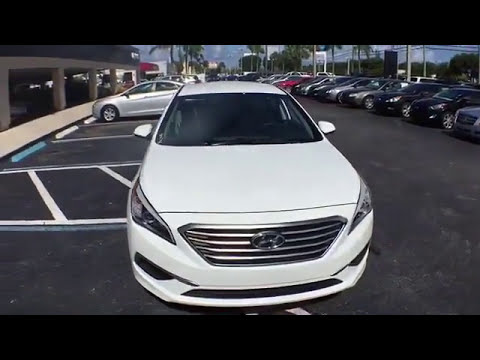The photograph features a detailed image of the front end of a white Hyundai sedan, seemingly captured in a parking lot. The sedan is positioned almost directly facing the camera, revealing its hood, grille with the Hyundai logo, windshield, and roof, along with its white side mirrors. The parking lot surface appears dark gray or nearly black. The photo has a small rectangular shape with thick horizontal black borders at the top and bottom. In the background, there are multiple other parked cars, indicating the car is part of a larger array of vehicles in the lot. Some white lines denoting parking spaces are visible, with a notable blue stone curb marker indicating a handicapped spot. The background also includes a few palm trees and a bit of sky, which has a grayish-blue hue. There is a building to the left side, which might be part of a parking garage, adding to the urban setting vibe of the scene.